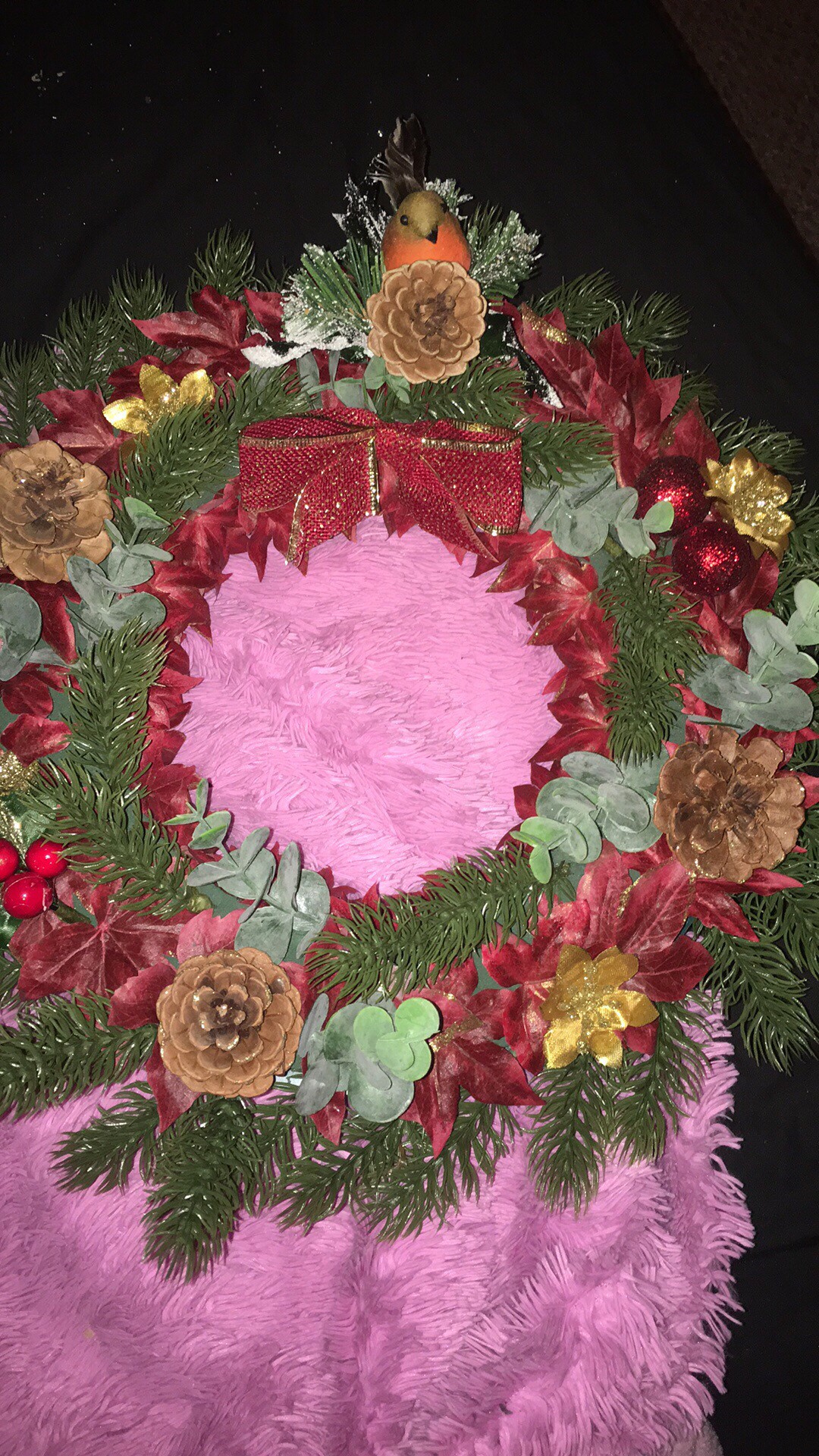This photo features a holiday-themed, circular Christmas wreath approximately 12 inches in diameter. The wreath itself is lush green and adorned with several festive decorations: glittering red balls, gold faux flowers, brown pine cones, and a bright red bow with gold trim situated at the top center. There's also a dusting of artificial snow and sprigs of plastic holly berries, adding to the seasonal charm. The wreath appears to include a small decorative bird with orange and light brown hues perched near the top. Surrounding the wreath is a fluffy purple fabric, possibly a shawl or blanket, set against a black background, creating a striking contrast that highlights the vibrant colors of the wreath.